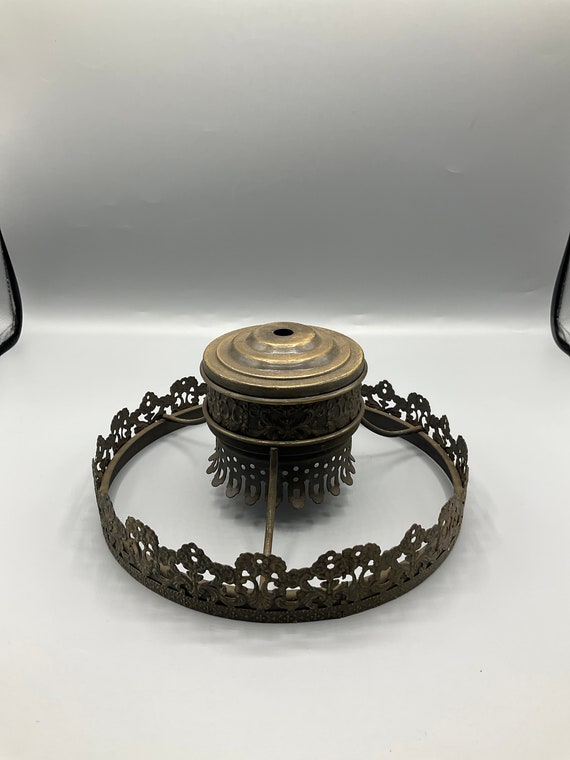This image showcases a cylindrical metal object, likely part of an antique lantern or lamp, set against a plain white background. The object has a dull brass or copper hue and intricate designs, featuring patterns resembling stylized trees or flowers around its middle and outer rim. The cylindrical part has a top hole and extends downward into a base adorned with petal-like extensions. Three metal prongs radiate outward from the center to connect to the outer rim, incorporating the same tree-like designs, adding a decorative and functional element to the structure. The object's precise size is unclear due to the close-up nature of the shot, but it stands on a solid white floor or desktop with a curved wall behind it. This appears to be a carefully crafted, ornamental piece of a lighting device from an earlier era.